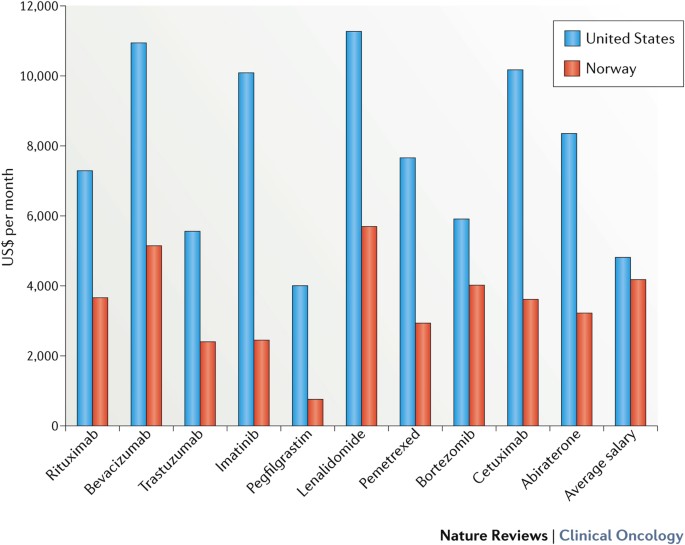The image is a detailed bar graph from the journal "Nature Reviews Clinical Oncology," specifically under the "Nature Reviews" section. The graph compares the monthly expenditure in US dollars on various medications between the United States and Norway. Medications listed include Rituximab, Bavaxixumab, Trastuzumab, Imatinib, Pegfilgrastim, Lenalidomide, Pemetrexed, Bortezomib, Cetuximab, and Abiraterone, as well as the average salary. The United States, represented by blue bars, consistently shows higher spending than Norway, represented by red bars, with expenditures ranging from zero to twelve thousand dollars per month on the y-axis. The x-axis lists medication names in what appears to be Norwegian. The overall visual is dominated by the significant spending disparity, with U.S. bars often rising two to three times higher than those of Norway.